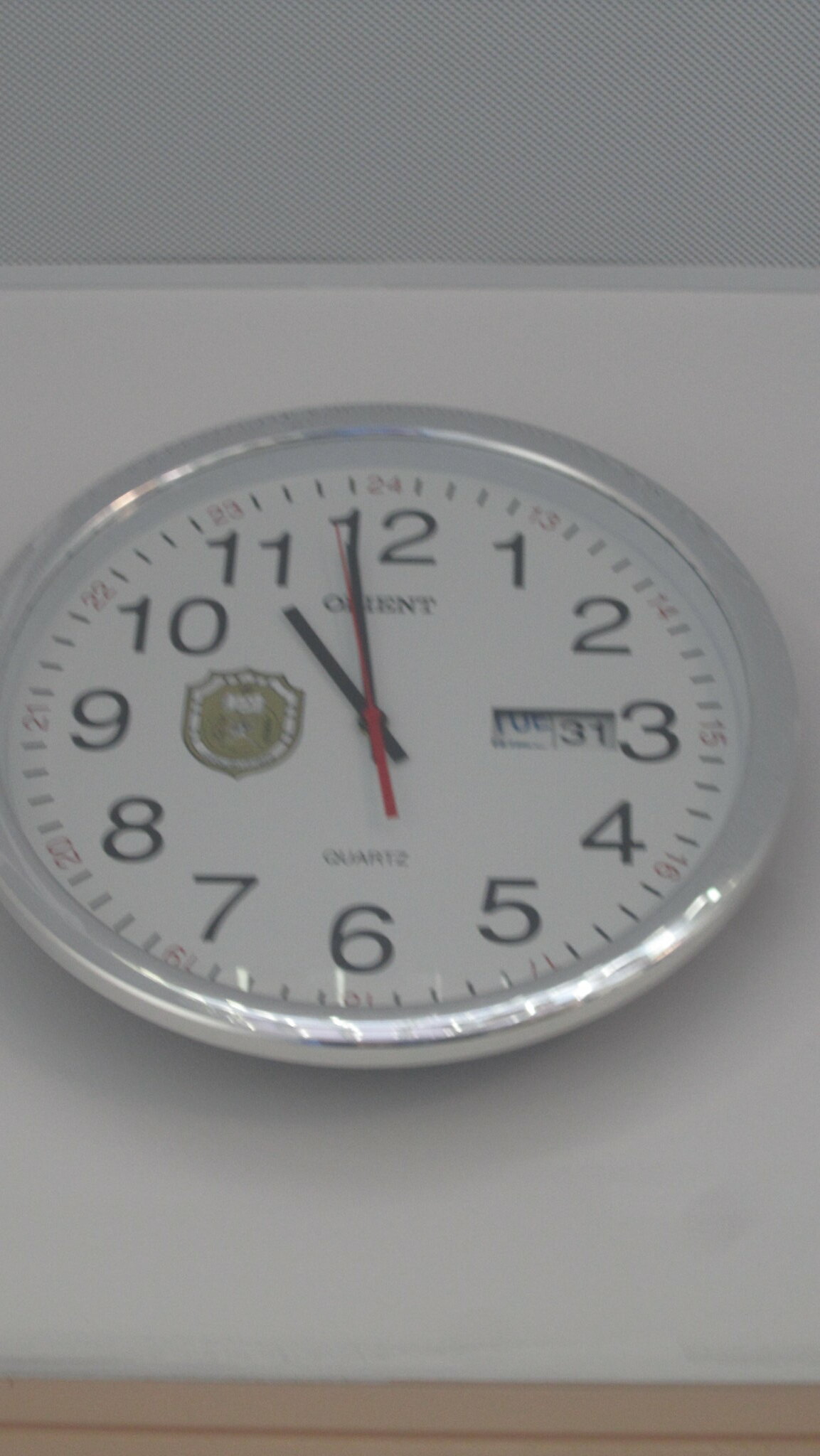This photograph features a close-up view of a round wall clock, slightly tilted from below looking upwards. The background is predominantly white, transitioning to a grayish tone near the top edge, with a narrow brown strip running along the base of the wall. The clock is almost centrally positioned in the photograph, but its left edge is partially cropped out of the frame.

The clock has a silver metallic rim and a white face with black numbers ranging from 1 to 12. The time is approximately 11:58, indicated by the short black hour hand, long black minute hand, and a very long, thin red second hand. At the 9 o'clock position, there is a blurry symbol resembling the outline of a police badge in light green. Adjacent to the 3 o'clock position is a date window displaying "Tuesday the 31st." Additionally, the word "quartz" appears above the 6, and another indistinct word is present beneath the 12. The photograph's slight angle introduces a mild distortion to the clock's shape, contributing to its imperfect sharpness.